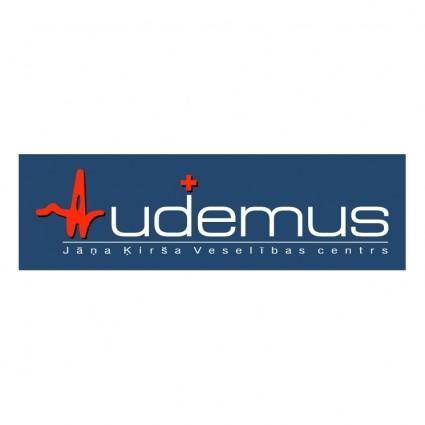The image is a computer-generated graphic featuring a rectangular blue sign, primarily in a dark blue hue. Prominently displayed on the left side of the sign is a red symbol resembling an EKG heartbeat line—a zigzag pattern with a triangular peak followed by another zigzag. Adjacent to this symbol is the text "udemus" in lowercase white letters, with a red cross or plus sign positioned directly above the letter "d." Below this text, a thin horizontal white line stretches across the sign. The words "janakirasveseltbas centers" are written underneath the line in white text, with no additional imagery or people present in the image.